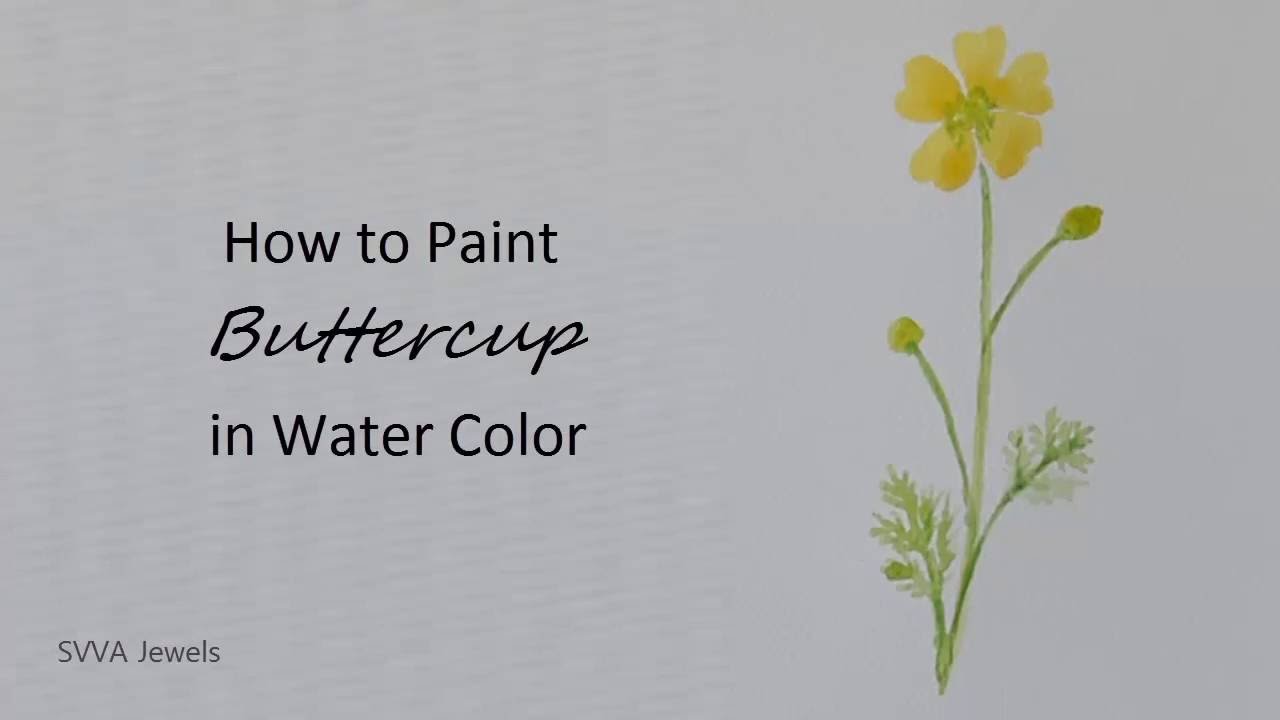This image resembles a title slide for a YouTube tutorial video. The background is predominantly grey, with the left side featuring faint, slightly darker diagonal lines creating a subtle, ridged pattern. On the left half of the image, centered black text reads "How to Paint Buttercup in Watercolor," with the word "Buttercup" written in a cursive script. At the bottom left corner, small black text states "SVVA Jewels." To the right side of the image, there's a watercolor illustration of a buttercup flower. The illustration showcases a tall green stem with offshoots; at the bottom, two leafy sprigs, and in the middle, two buds that have yet to bloom. At the very top of the stem, there is a yellow-petaled buttercup flower with a greenish center. This entire design is set against a grey backdrop, emphasizing the delicate artistry and instructional nature of the content.